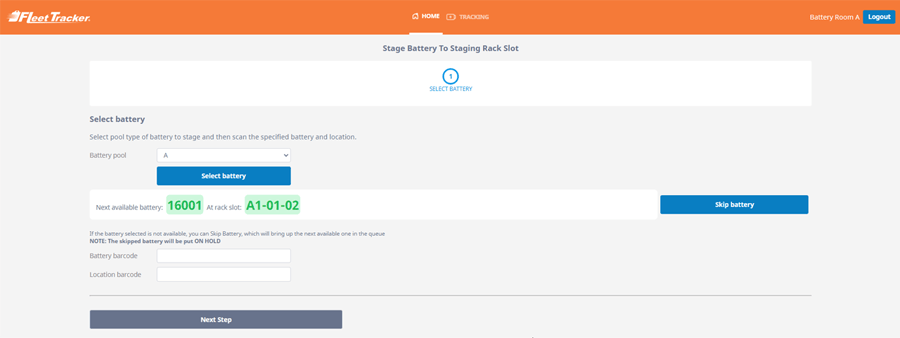The image depicts a computer screen with a layout that is long and narrow. At the top, an orange band stretches across the screen and contains various elements. 

On the left-hand side of this orange band, the text "Fleet Tracker" is prominently displayed. In smaller type on the far left, the word "Home" is shown, and next to it, partially obscured text that likely reads "Tracking." On the right-hand end of the orange bar is an option labeled "Log Out."

Below the orange bar, the screen is predominantly gray. At the top of this gray section, the text "Stage Battery to Staging Rack Slot" is evident. Beneath this heading, a blank white box contains a blue icon with the text "Select Battery." 

In black text just below this box, instructions appear that prompt the user to "Select Battery.” These instructions further detail that the user should select a type of battery to stage and then scan the specified battery and its location. 

Further down, another section labeled "Battery Pool" appears, from which the user can select a battery. Here, a white box displays the text "Not Available Battery.” Directly below, it indicates that the next available battery is "16001 at Rack Slot A1-01-02." Additional unspecified information follows this, offering the option to either use this specific battery or skip it and select another. The details about the location are also noted but not fully described within the view of this screen.